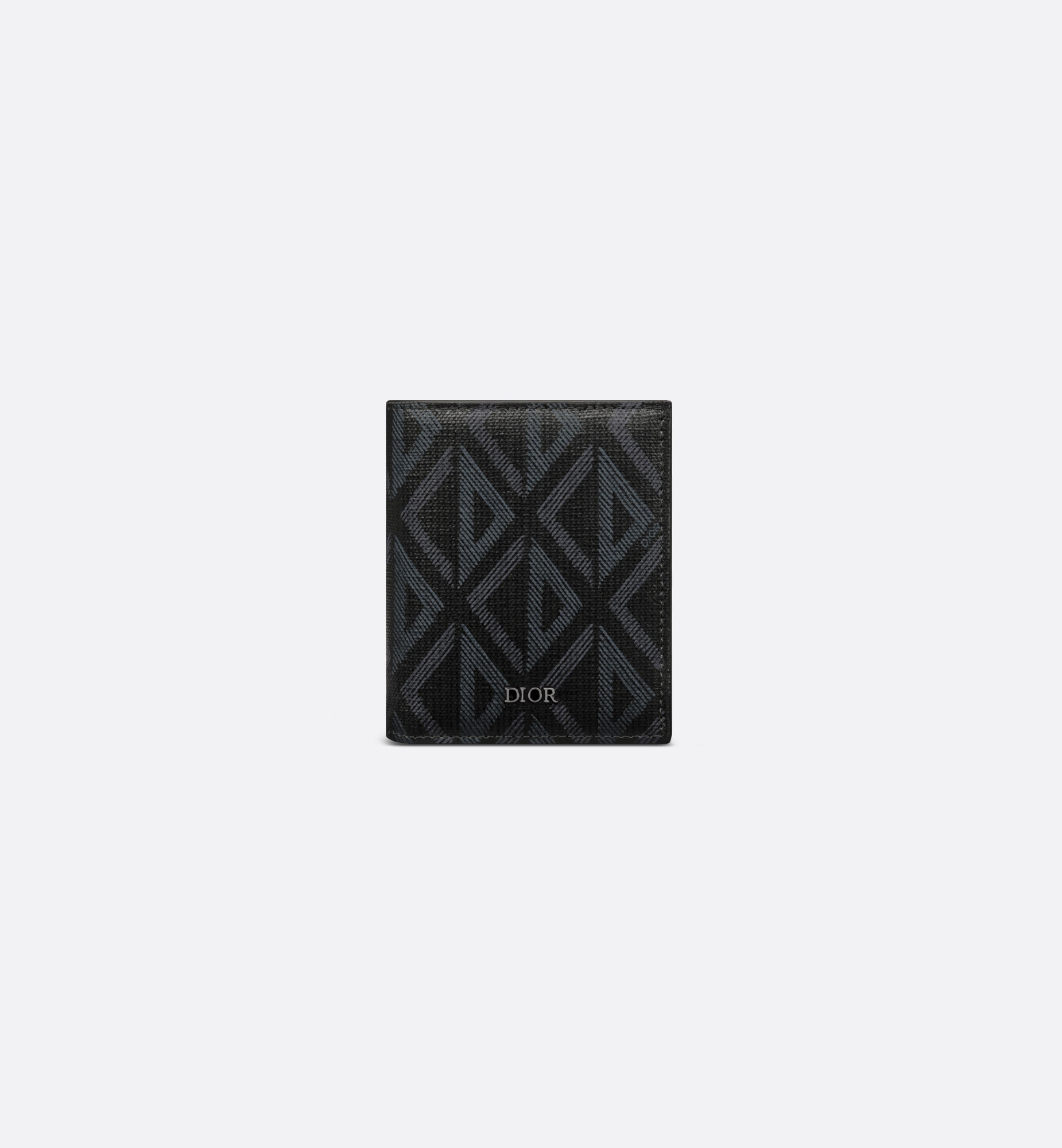The photograph features a luxurious Christian Dior wallet, prominently centered against a plain white background. The wallet, likely crafted from leather, boasts a sleek, folded design. It is predominantly black, accented with dark grey and white details that contribute to its sophisticated appearance. The distinctive Dior logo, etched in light grey, is positioned elegantly at the bottom. Additionally, the wallet is decorated with geometric patterns resembling triangles and the letter 'C', creating a subtle yet refined motif. White stitching frames the edges, reflecting the meticulous craftsmanship synonymous with the Dior brand. This detailed image, with its emphasis on high-quality materials and impeccable design, evokes the elegance and luxury one would expect when shopping for premium fashion accessories online.